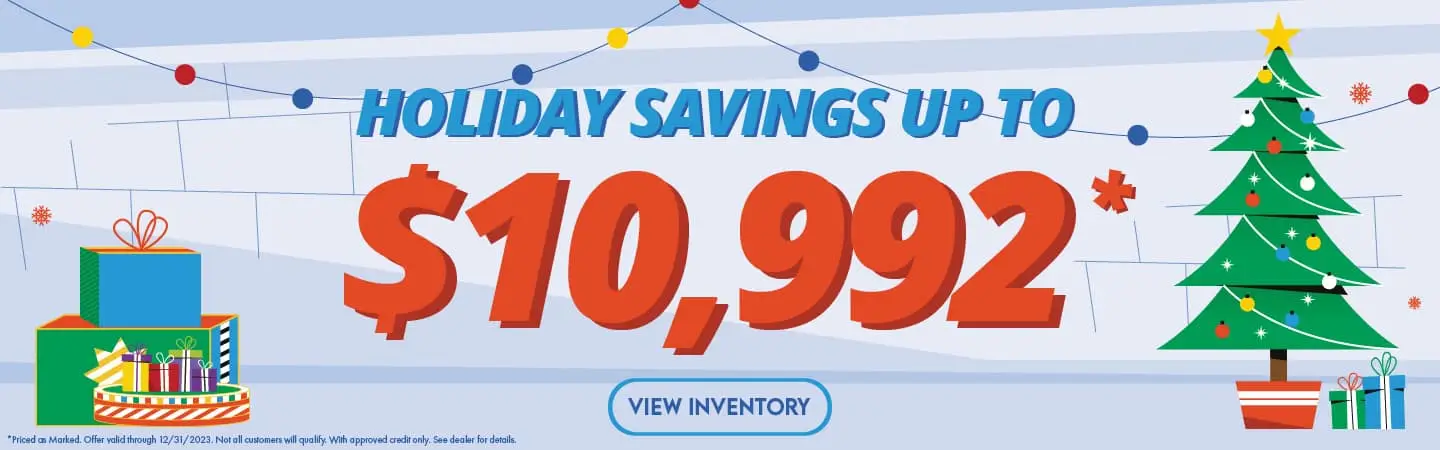**Holiday Savings Sale Banner Advertisement**

This rectangular holiday-themed advertisement measures approximately seven inches wide by one to two inches tall. At the center, the text prominently reads, "Holiday Savings: Up to $10,992," followed by an enticing call-to-action that states, "View Inventory." This suggests it is part of a website's promotional campaign, perhaps to entice customers to explore holiday deals on various items.

The scene is festive and vibrant, with a cartoonish Christmas tree on the right side. The tree is adorned with colorful ornaments and a shining star at the top. It stands in a decorative red and white tree stand, surrounded by a few wrapped presents – one in blue paper and another in green with a bow, adding to the festive spirit.

Above, a string of Christmas lights is hung across the top of the image, looping elegantly in the center to evoke a cozy holiday atmosphere. On the left side of the banner, additional presents are visible, further enhancing the holiday shopping theme of the advertisement.

The overall composition clearly indicates that this banner is designed to promote pre-Christmas sales, encouraging viewers to take advantage of substantial savings as they shop for gifts.